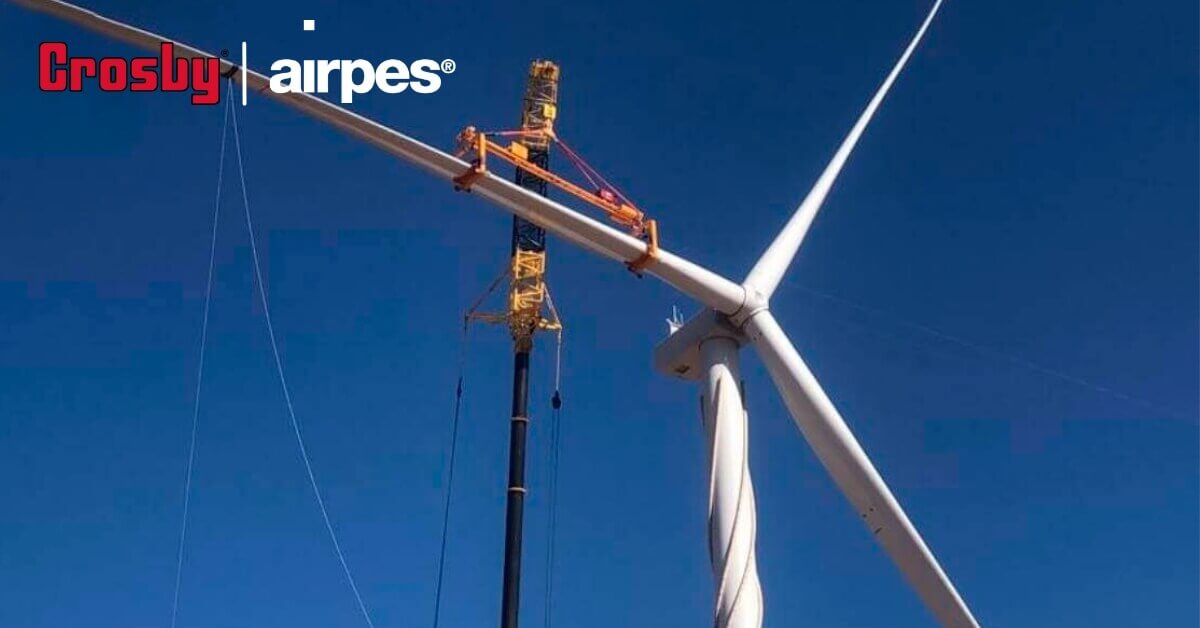In this dynamic outdoor scene, a white wind turbine gleams under a sunlit blue sky, transitioning from deep blue at the top to a lighter blue at the bottom. The turbine features three large blades radiating from the center: one angle up to the top left, another off-center to the top right, and the third stretching down to the bottom right. Prominently, the top left corner displays the bold red logo "Crosby" in capital letters, followed by the name "Airpes" in white block letters with a registered trademark symbol. Adjacent to the turbine, a yellow crane with black segments and dangling wires is attached to one of the blades, suggesting maintenance or assembly work. Beside the crane, a tall black pole with white stripes runs vertically, adding complexity to the structure with additional wires suspended in the air, enhancing the technical essence of the scene.